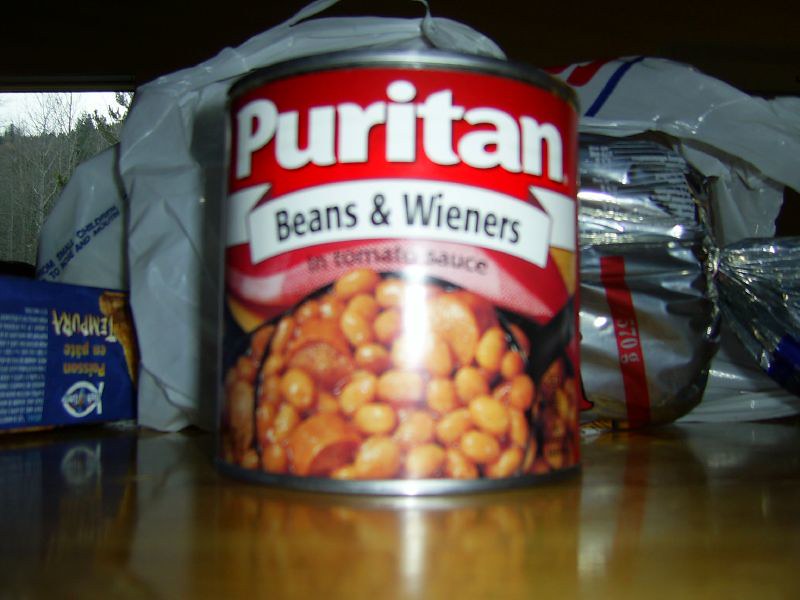This is a horizontal, close-up photograph of a light brown wooden table with a central focus on a can of "Puritan Beans and Wieners in Tomato Sauce." The can features a red banner with the word "Puritan" in white letters, a white banner with "Beans and Wieners" in black letters, and a pink banner stating "In Tomato Sauce." The label includes a photo of beans and cut-up hot dogs, or wieners, as described. Behind the can, there is a silver and red loaf of bread partially visible inside a grocery plastic bag. To the left, you can see a blue box labeled "tempura" with some text in French, which is partly obscured and upside down. The background includes a view of a window and trees, indicating that the setting might be outdoors but under some covering. The image’s focus is partly out of depth, emphasizing the can while slightly blurring the surrounding items.